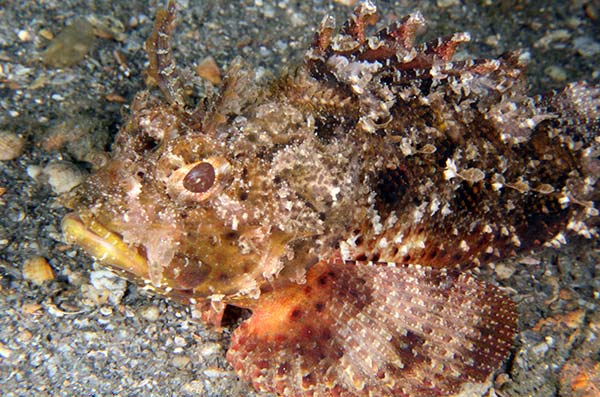This close-up color photograph features a heavily camouflaged fish that blends seamlessly with its rocky background. The fish, likely a type of rockfish, exhibits a complex pattern of spots in brown, white, yellow, orange, and some hints of black. Its stout body, covered in rough, rock-like scales, enables it to disappear into the surrounding stones and gravel, which are predominantly whitish-gray. The fish has notable pink eyes, which resemble round stones, and its large mouth remains closed. Its prominent front fins and a slightly shorter tail fin further mimic the shapes and colors of rocks and shells around it. The image's indistinct background, which could be the bottom of an aquarium, stream, lake, or ocean, is filled with similar stones and sand, enhancing the fish's camouflaged appearance. The fish is glancing to the side, presenting a vigilant, almost stern expression with its brown eyes. The overall visual effect is one of masterful disguise, as the fish merges nearly indistinguishably with its environment.